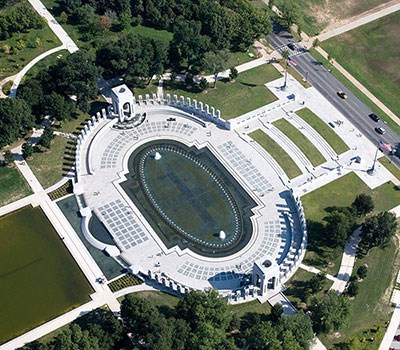This image presents an aerial view of an oval-shaped stadium that resembles a Colosseum. The stadium is in poor condition and notable for its four spectator areas colored white. The central green field is also deteriorated, featuring two white objects at one end. At the far corners of the stadium, two towers can be seen, encased by what appears to be a surrounding fence. The scene is dominated by shades of white and green, spotlighting the bright sunlight typical of daytime.

To the right side of the stadium, there are three rectangular patches of grass, bordered by white paths, leading towards a three-lane road with cars traveling on it. The background is enriched with green vegetation, including clusters of trees, adding a natural contrast to the concrete structure. The configuration of the image places the stadium centrally, stretching diagonally from the top left to the bottom right corner, with the adjacent road and greenery enhancing the overall perspective.